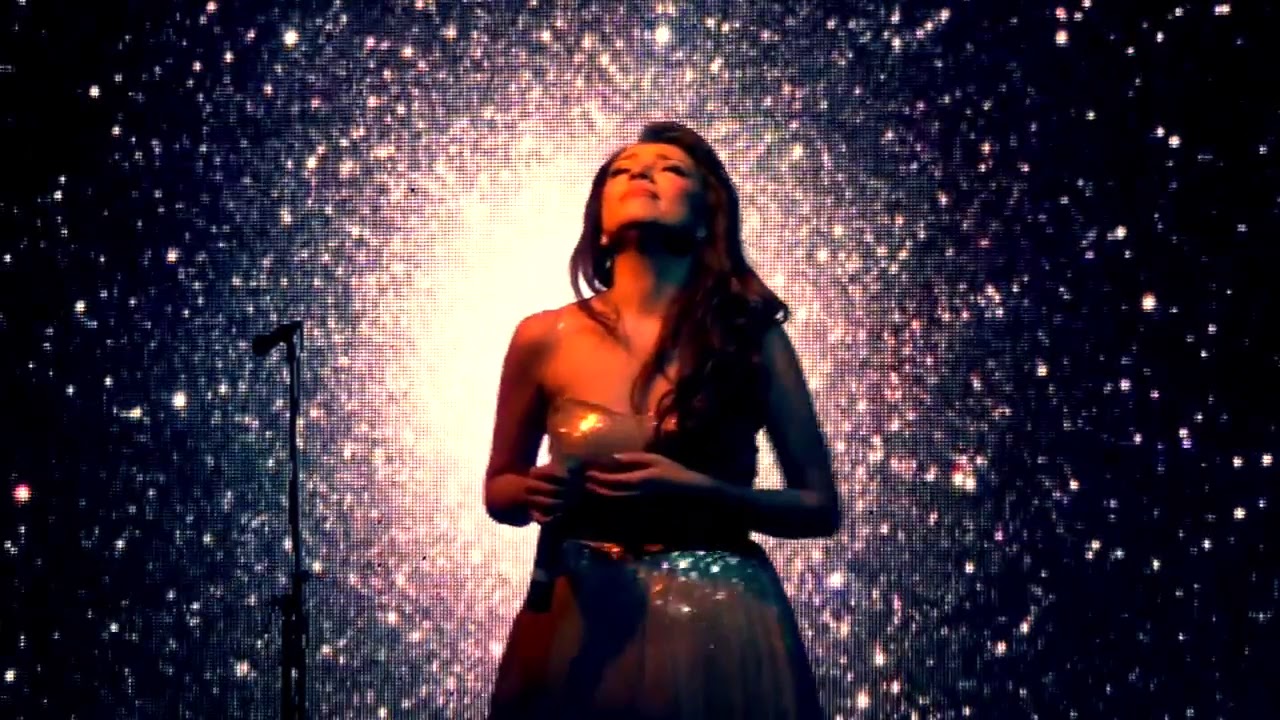In the image, a woman stands at the center, bathed in the dramatic light of a powerful, radiant explosion behind her that illuminates the scene, casting brilliant white luminescence outward against a pure black background. The light source, resembling a 'big bang,' features sparkles that gradually darken as they spread. The woman is adorned in a sparkly, silvery dress with thin straps, and she holds a candle close to her chest, emitting a warm orange glow onto her serene face. Her long dark hair cascades around her as her eyes remain closed in peaceful contentment, her lips curved in a slight smile. A microphone stand is positioned to her left, indicating she might be a performer, further highlighted by her poised stance and the ethereal backdrop that frames her.